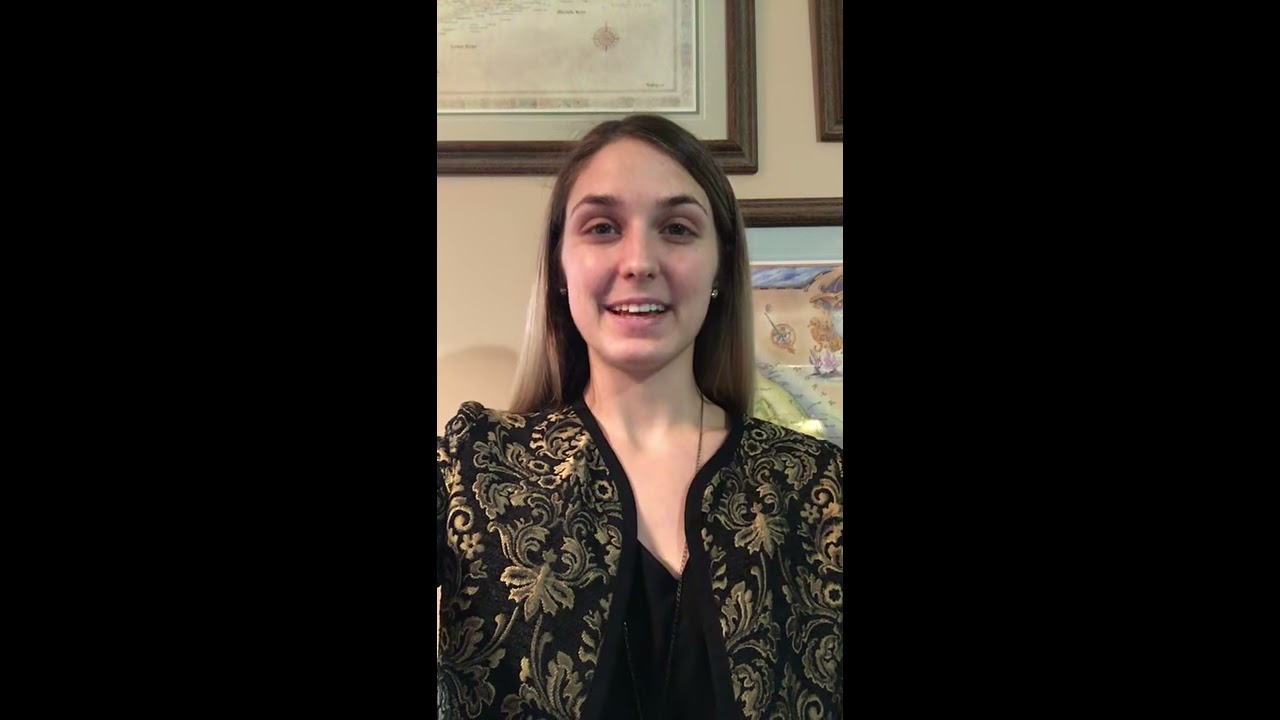The photograph features a Caucasian woman in her late 20s with long, dark hair accented by sandy blonde highlights. She is smiling broadly, showing her teeth without grinning, and looking directly at the camera, emanating a sense of warmth and friendliness despite her slightly tired eyes accentuated by subtle eye makeup. The woman is wearing large stud earrings and a long chain necklace that extends down but is partially obscured by her attire. Her outfit consists of a black top and a striking, Victorian-inspired black jacket adorned with intricate gold filigree, which includes detailed foliage and possibly moth designs. The jacket features a distinctive black neckline and lacks buttons, opening at the center. 

The setting appears to be indoors, against a taupe-colored wall decorated with three framed items – possibly academic certificates or artwork – in brown wooden frames, one of which is partially obscured by her head. The frames behind her include one colorful piece. The entire image is divided by solid black panels on both the left and right sides, framing the central image of the woman, who is positioned towards the bottom center of the frame. The style of her clothing suggests the photograph was taken within the last seven years, given the blend of vintage and contemporary elements.